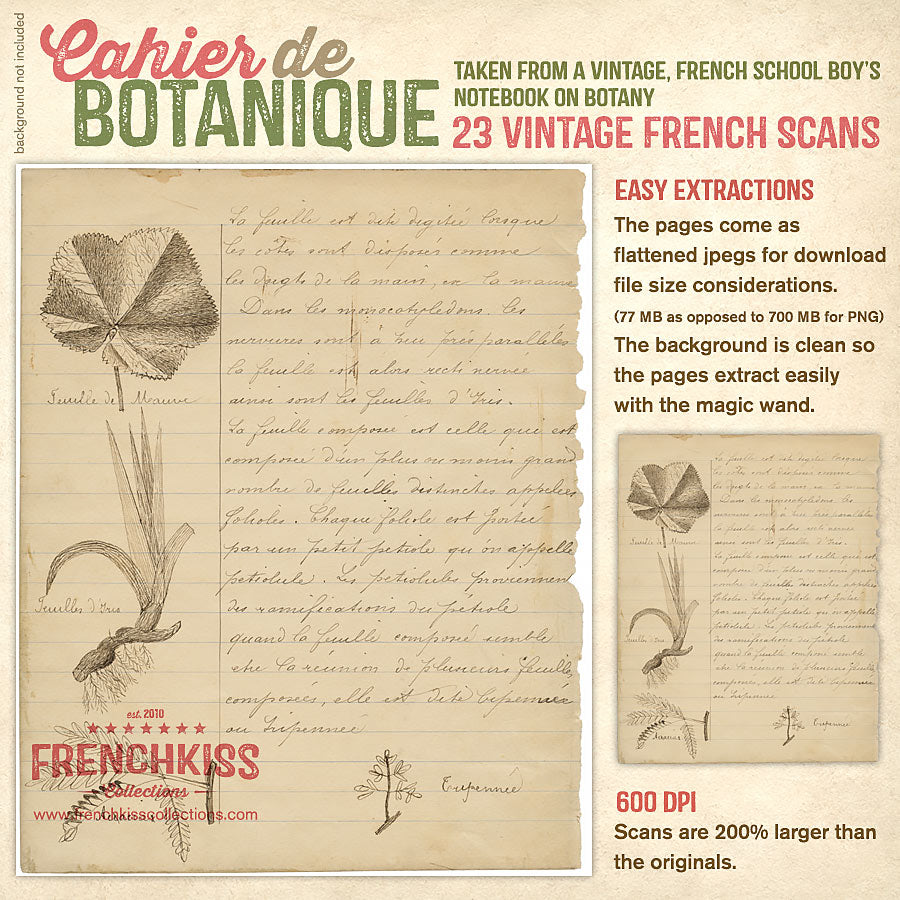This detailed infographic, titled "Cahiers des Botaniques," presents a collection available for download from French Kiss Collections, established in 2010. The image has a tan background and features a mix of French and English text. "Cahiers" is in red, "des" in gray, and "Botaniques" in green, with most of the other text also in green or red. 

Promoting "23 French scans" taken from a vintage French schoolboy's notebook on botany, the infographic emphasizes easy extractions due to clean backgrounds that work well with the magic wand tool. The downloadable pages come as flattened JPEGs, making them significantly smaller in file size (77 MB) compared to PNGs (700 MB). 

The left side of the image includes text like "easy extractions" in red, and towards the bottom, it notes that the high-quality 600 DPI scans are 200% larger than the originals. On the right-hand side, there's an inset image of a hand-drawn flower with frayed notebook edges, suggesting authenticity and age. Below this main image is a smaller close-up inset featuring hand-drawn details of leaves and grass with roots. 

Additional French handwritten notes appear on the far left, contributing to the vintage botanical theme. The branding feature at the bottom of the infographic is "French Kiss Collections," along with its establishment year of 2010. The image gives a clear example of the downloadable content, making it clear that the collection is both a practical resource and a historical homage.